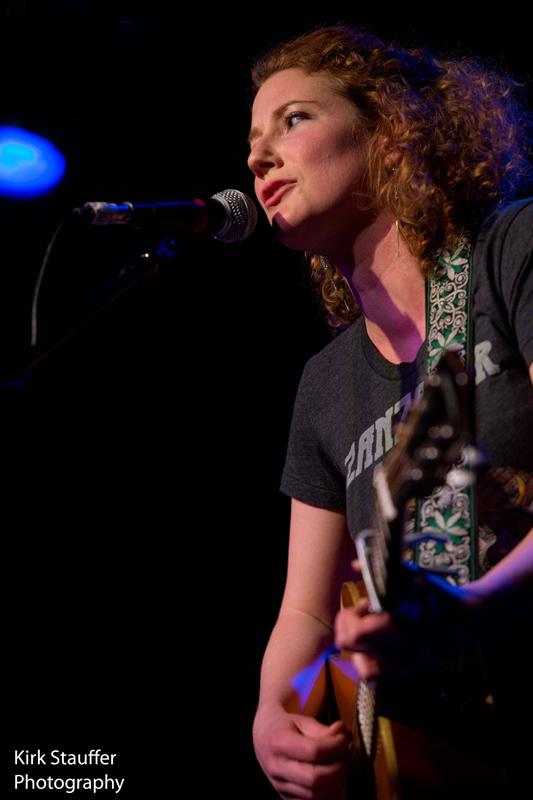This is a color photograph in portrait orientation featuring a woman on stage, captured from the top of her head to about her waist. She has curly, reddish-brown hair and some freckles on her face. The woman is singing into a silver microphone with a blue handle positioned to the left of her mouth while strumming a brown acoustic guitar with her right hand. Her attire includes a black t-shirt with the partially visible text starting with "ZAN" and a green guitar strap adorned with a white floral design over her shoulder. A blue light in the top left corner illuminates her, and the background is predominantly black. In the bottom left corner, there is a small white text credit that reads "Kirk Stauffer Photography."